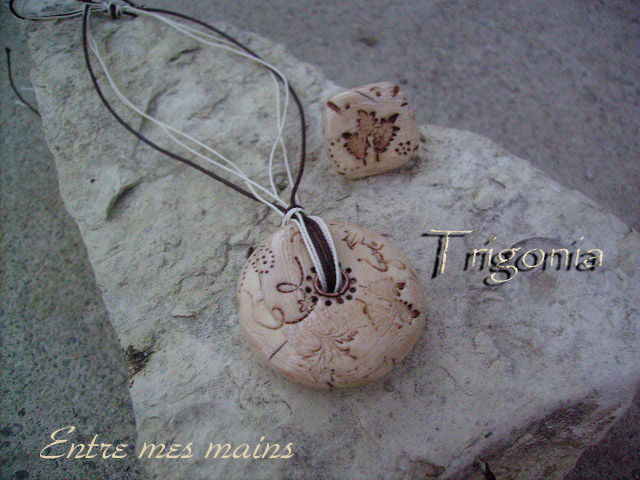The image depicts a triangular stone positioned on a gravelly stone surface, with its tip pointing to the upper left corner and its base facing the bottom right of the image. Resting upon this triangular stone is a circular string necklace with alternating white and dark brown threads. The circular pendant of the necklace is light brown, decorated with intricate designs of leaves, flowers, and stars. Adjacent to the necklace, towards the left, is a square ornament that shares the same color and features a pattern of three leaves. Both the necklace and the square ornament appear to be made from a hard material, possibly wood or stone, and exhibit a vintage and antique style. In the top right corner of the image, the text "Chai Ga Near" can be seen, while "Ender Mist Minks" is inscribed at the bottom right. Additionally, other text on the triangular stone reads "Trigonia," with 'Trigonia' separated, and below it, in cursive, "Entrez mains." The overall aesthetic suggests an outdoor setting, potentially evoking the impression of fossils or ancient artifacts.